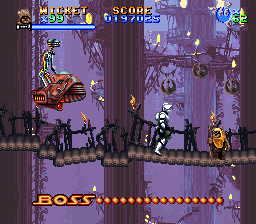The image is a screenshot from what appears to be a retro 80s-style video game set in a purple-hued dystopian fantasy world. Dominating the center is a large treehouse, part of a treetop village connected by wooden plank walkways and log bridges. Wicket W. Warwick, an Ewok from Star Wars, is the main character visible on a rickety log bridge with broken ropes. He holds a flaming torch, and beside him, there is a biker scout from the original Star Wars films. 

In the top-left corner, "Wicket x 99" possibly indicates the character's health or power level, accompanied by a score display. At the bottom of the screen, the word "BOSS" is prominently displayed in large, bold yellow letters followed by dots, suggesting this scene is a boss level. To the right, in mid-air, stands a robot-like creature on a flying vehicle resembling a moped, likely the boss Wicket must defeat. The background is richly detailed with additional massive trees, emphasizing the Ewok village setting high among the treetops.